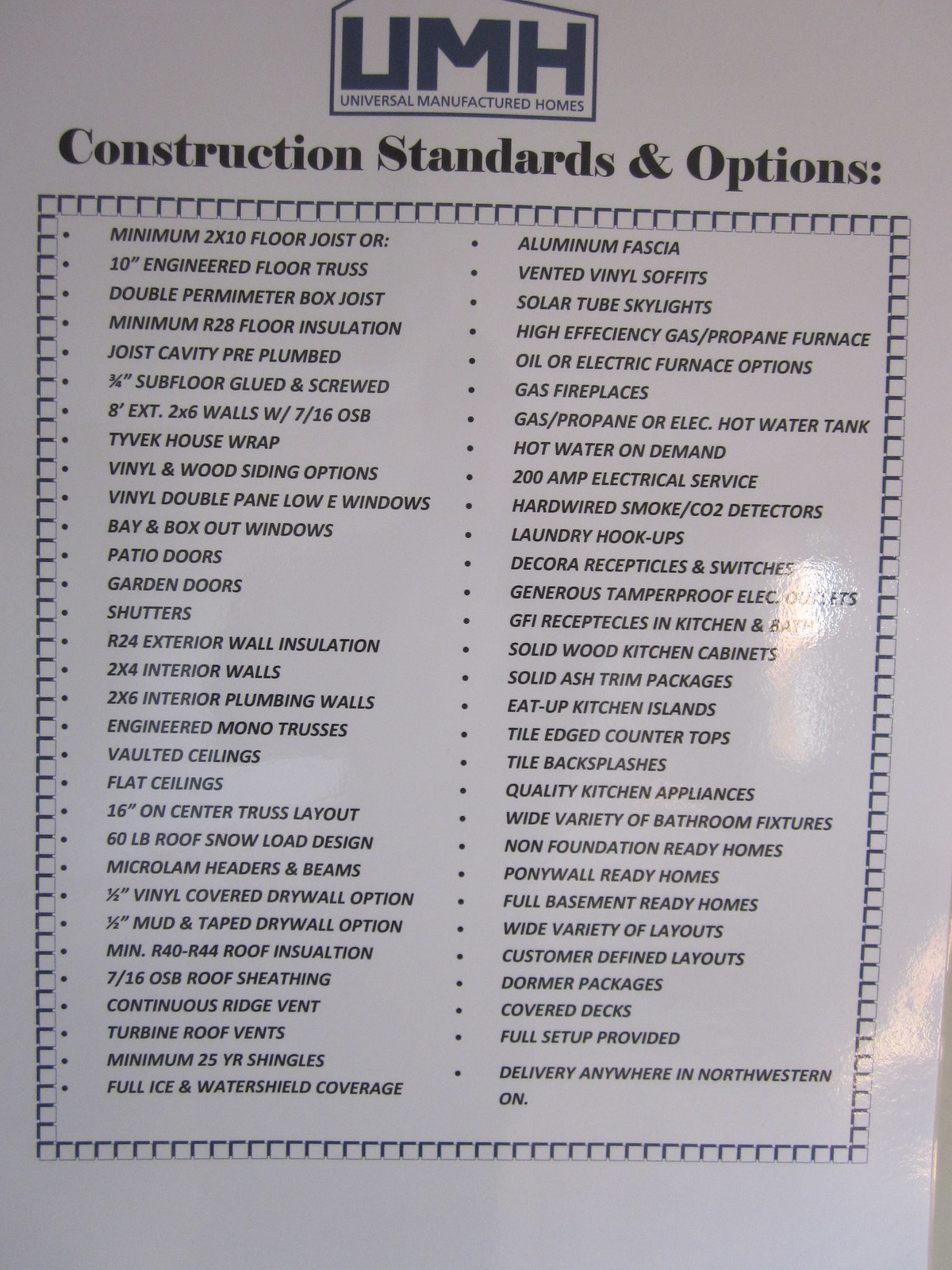The advertisement for Universal Manufactured Homes features a pristine white background with a distinguished blue outline of a house in the upper middle section. Prominently displayed in bold blue uppercase letters, "UMH" stands out above the company name, "Universal Manufactured Homes." Just below, it reads "Construction Standards and Options" in a dark black font. The entire layout is framed by blue squares, emphasizing the core information in the center of the paper.

The extensive list of construction standards and options includes crucial specifications such as a minimum of 2x10 floor joists or 10-inch engineered floor trusses, double perimeter box joists, minimum R28 floor insulation, joist cavity pre-plumbed, and 3/4-inch subfloor glued and screwed. The document highlights robust construction features like 8-inch exterior 2x6 walls with 7/16 OSB, Tyvek house wrap, options for vinyl and wood siding, vinyl double-pane low-E windows, bay and box-out windows, and patio and garden doors.

Additionally, it lists R24 exterior wall insulation, 2x4 interior walls, 2x6 interior plumbing walls, engineered roof trusses, vaulted or flat ceilings with a 16-inch on-center truss layout, and micro-laminated header beams, all designed to ensure durability and comfort. The options also promise high-quality finishes with garden doors and shutters, offering customizability alongside standard features. Delivery is available anywhere in Northwest Ontario, accommodating a wide geographic range.